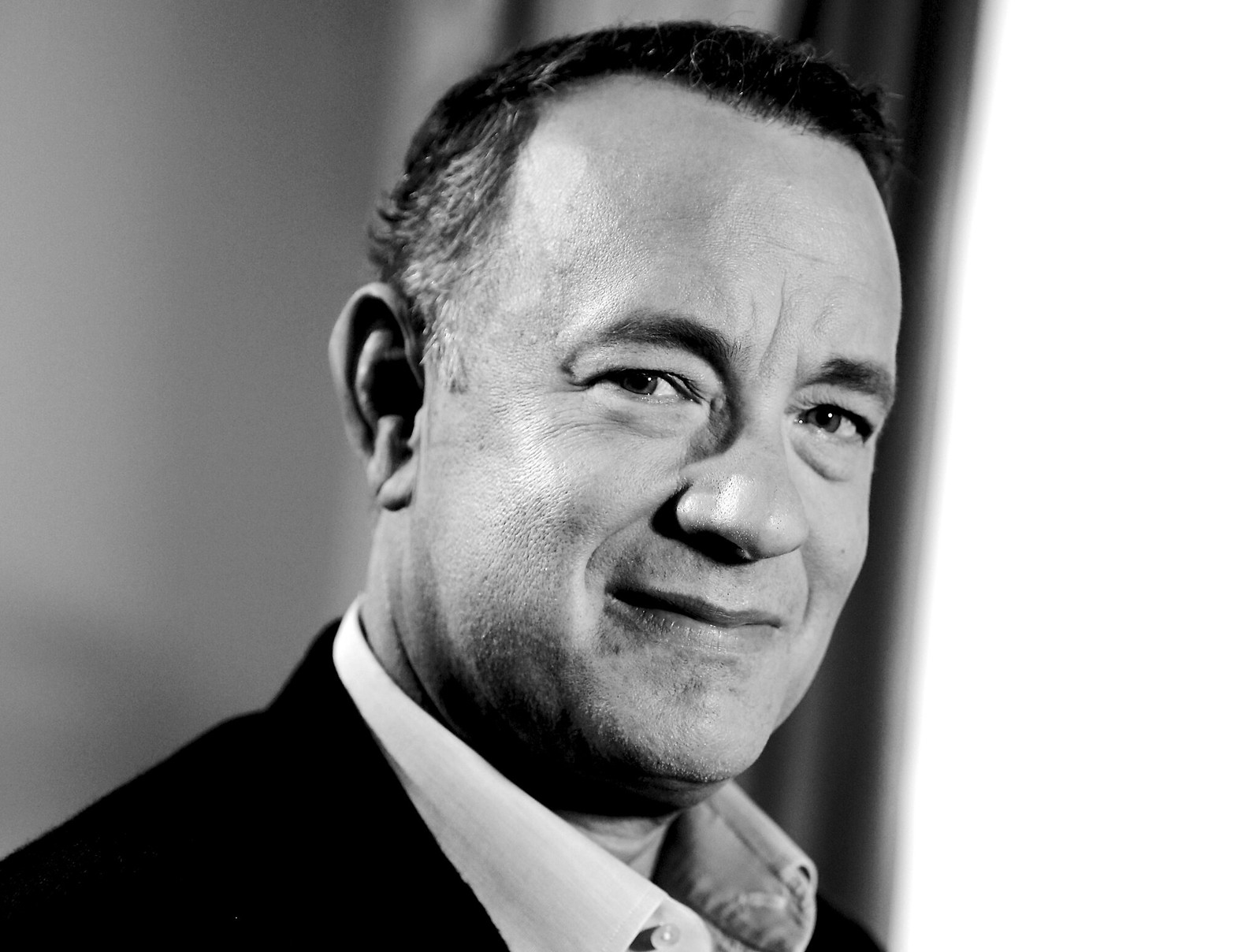This vintage black-and-white photograph features a young Tom Hanks smiling subtly at the camera. He is dressed in a dark suit over a white, open-collared button-up shirt, with no visible tie. His short hair is predominantly dark but shows a touch of gray on the sides. The backdrop appears somewhat ambiguous due to its blurred nature, but it includes what may be part of a curtain or a white wall, suggesting he is indoors, possibly in a room or a theater. The focus is primarily on Tom Hanks' face, capturing a clean-shaven, slightly stubbly look that accentuates his youthful appearance, estimated to be from around 20-25 years ago.